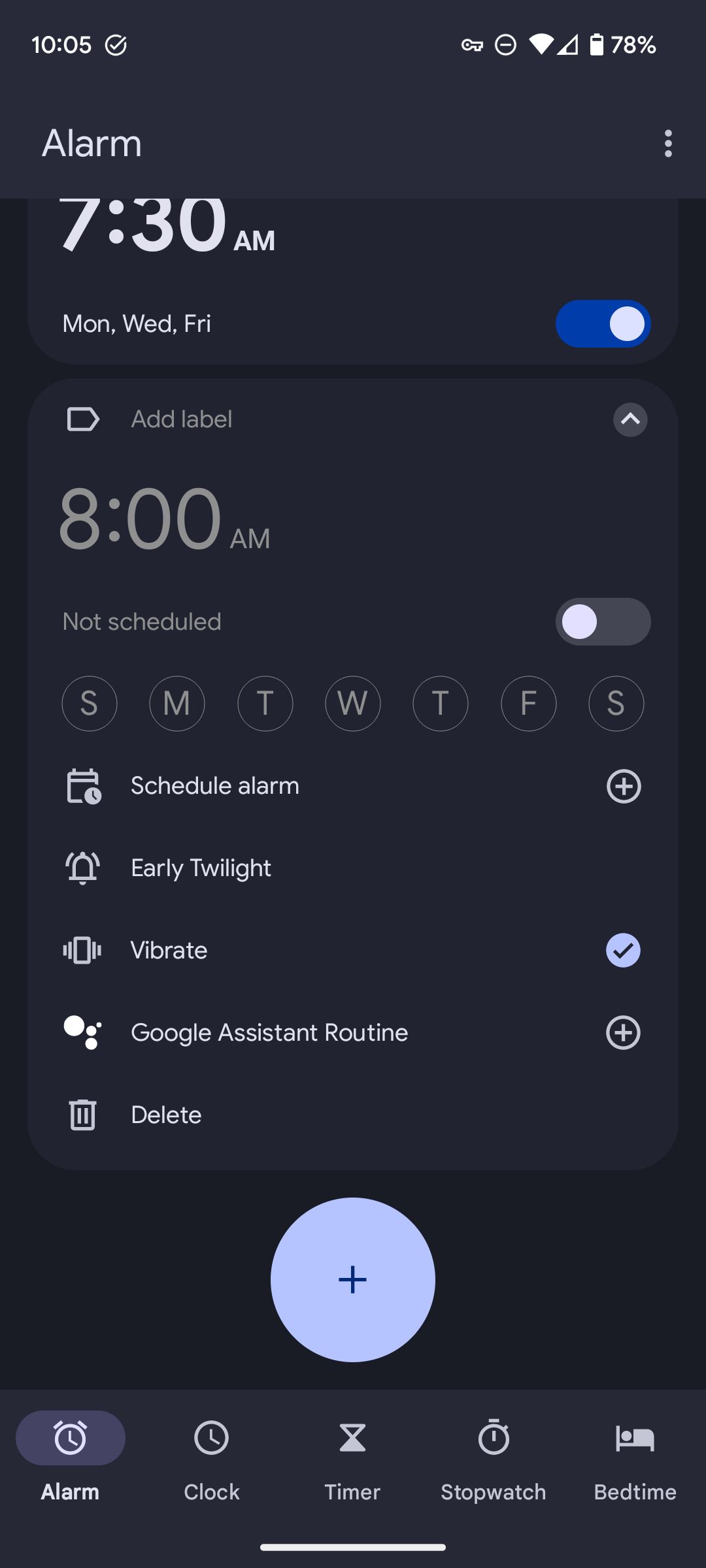The image is a mobile screenshot displaying an alarm settings page with a predominantly very dark grey and black background. At the top left of the screen, the word "Alarm" is clearly visible. Above this, in the header bar, the current time, various status icons, and a battery level indicator showing 78% are displayed.

The first alarm listed is set for 7:30 AM on Monday, Wednesday, and Friday, with a small active slider tab on the right, characterized by a white circle on a blue oval background, indicating it is turned on. The second alarm entry, positioned below, has the label "Add label" shown in a translucent font, signifying that this alarm is currently turned off. This alarm is set for 8:00 AM, but no specific days of the week are selected, and the slider tab for this alarm is turned off.

Directly beneath the second alarm, there are several functional icons with text beneath each, reading "Schedule alarm," "Early twilight," "Vibrate," "Google Assistant," "Routine," and "Delete," all in white font. Below these function icons, on the black background, is a light grey circle with a blue plus sign inside, suggesting an option to add a new alarm.

At the bottom of the screen, the footer contains five icons labeled "Alarm," "Clock," "Timer," "Stopwatch," and "Bedtime." The "Alarm" icon is highlighted with a small grey oval indicating it is the currently selected tab. Additionally, there is a thin horizontal white line at the bottom center of the image.